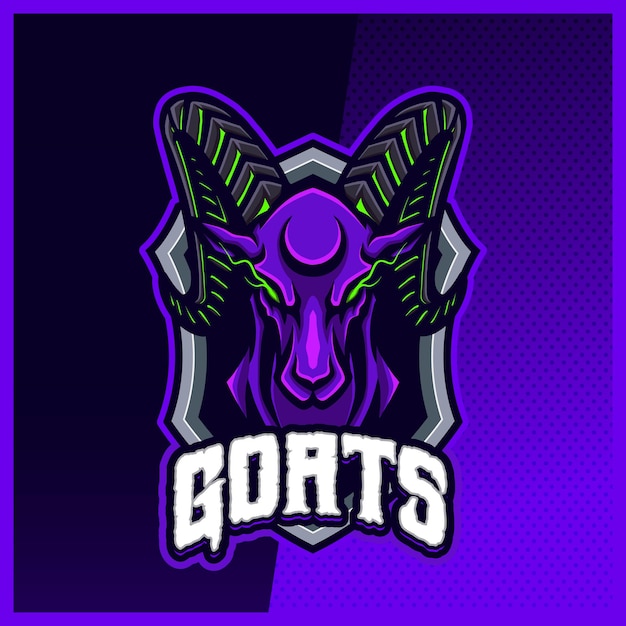The image depicts an eSports logo prominently displayed on a square canvas. The background is divided into two sections: the left side features a deep, dark purple while the right side transitions from a dark purple at the top to a lighter purple with a dotted pattern at the bottom. The entire image is bordered by a thin, purple outline.

At the center of the logo is a silver shield with a black interior. Positioned over the shield is a purple goat head with distinctive black and green horns. The eyes of the goat emit green lightning, and a black half-moon shape marks its forehead. Below the goat's head, the word "GOATS" is displayed in a bold, white block font accented by a purplish outline. The eSports logo exudes a dynamic and striking presence with its combination of vivid colors and intricate details.